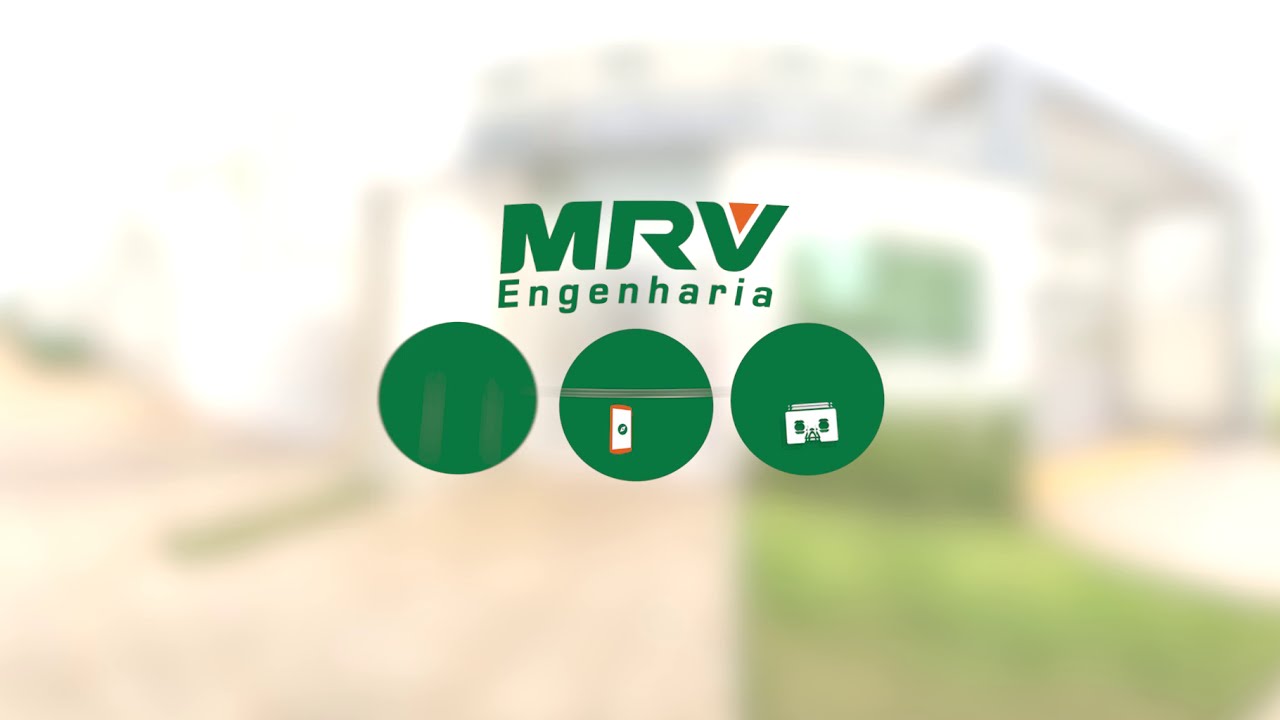The image is a horizontal, rectangular advertisement with a blurred background, giving an impression of a green yard interspersed with patches that could potentially be a brown roadway or a green and white building. Dominating the central portion, three horizontal rows of elements stand out. At the top, in large green letters, is "MRV," where the "V" features an orange triangle pointing downward at its center. The second row, also in green, reads "ENGENHARIA." Below these texts, there are three prominent green circles. The circle on the left is entirely solid green. The middle circle contains a few very light gray horizontal thin stripes just above the center, complemented by a vertical white rectangle with a red border located just beneath. This central circle bears a resemblance to a switch plate or smartphone icon. The circle on the right depicts a white and green outline of a building or house, featuring two vertical lines that could be windows near its top.